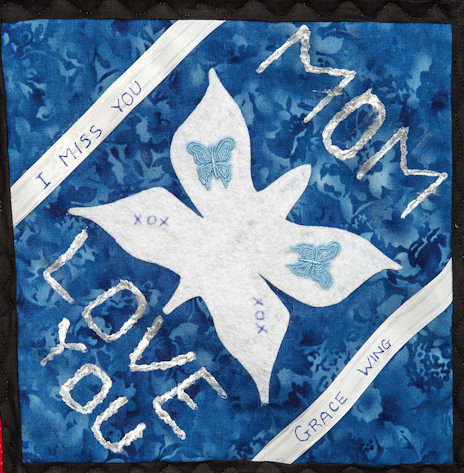The image displays a heartfelt, handcrafted piece of art on a multi-shaded blue, painted background, resembling a fabric-like texture. Central to the artwork is the handwritten word "Mom" in large, white letters, positioned diagonally across the top. Directly beneath, anchoring the bottom, it reads "love you," also in prominent white lettering. Nestled between these words is an artistic depiction of a white flower, possibly interspersed with elements that resemble butterflies, adding a delicate and loving touch.

Accentuating the edges, two white strips of painter's tape frame the composition. The strip at the top of the image bears the poignant message, "I miss you," written in blue pen, while the bottom strip carries the name, "Grace Wing," suggesting a personal and intimate connection. This detailed artwork appears to be a heartfelt token from a child to their mother, indicating love and longing, perhaps symbolizing a Mother's Day gift or a memorial tribute to a mother who has passed away. The use of colors such as black, white, light blue, dark blue, and silver enriches the visual appeal of this touching creation.